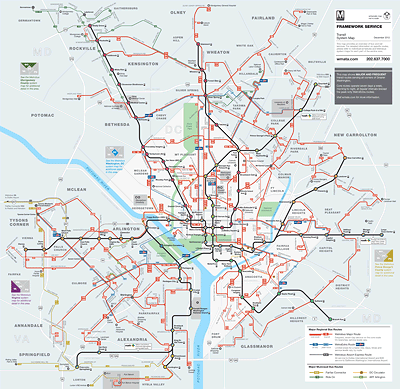This image is a map, likely representing metro and bus routes in the DMV area of Washington, D.C., Virginia, and Maryland. The map features various lines in black and red (or orange) that traverse the entire layout, suggesting transportation routes. A river runs from the left side down to the bottom center, branching into a Y shape as it moves up and to the right. The text on the map is very small and difficult to read, but a legend in the bottom right corner uses red, blue, and black to indicate different meanings. Additional explanatory diagrams are present in the top right portion, with one box in white containing red and black text, and another in dark gray with white text—both too small to decipher. The map presents a comprehensive view of public transportation in the specified area, overlaid on a light gray background.